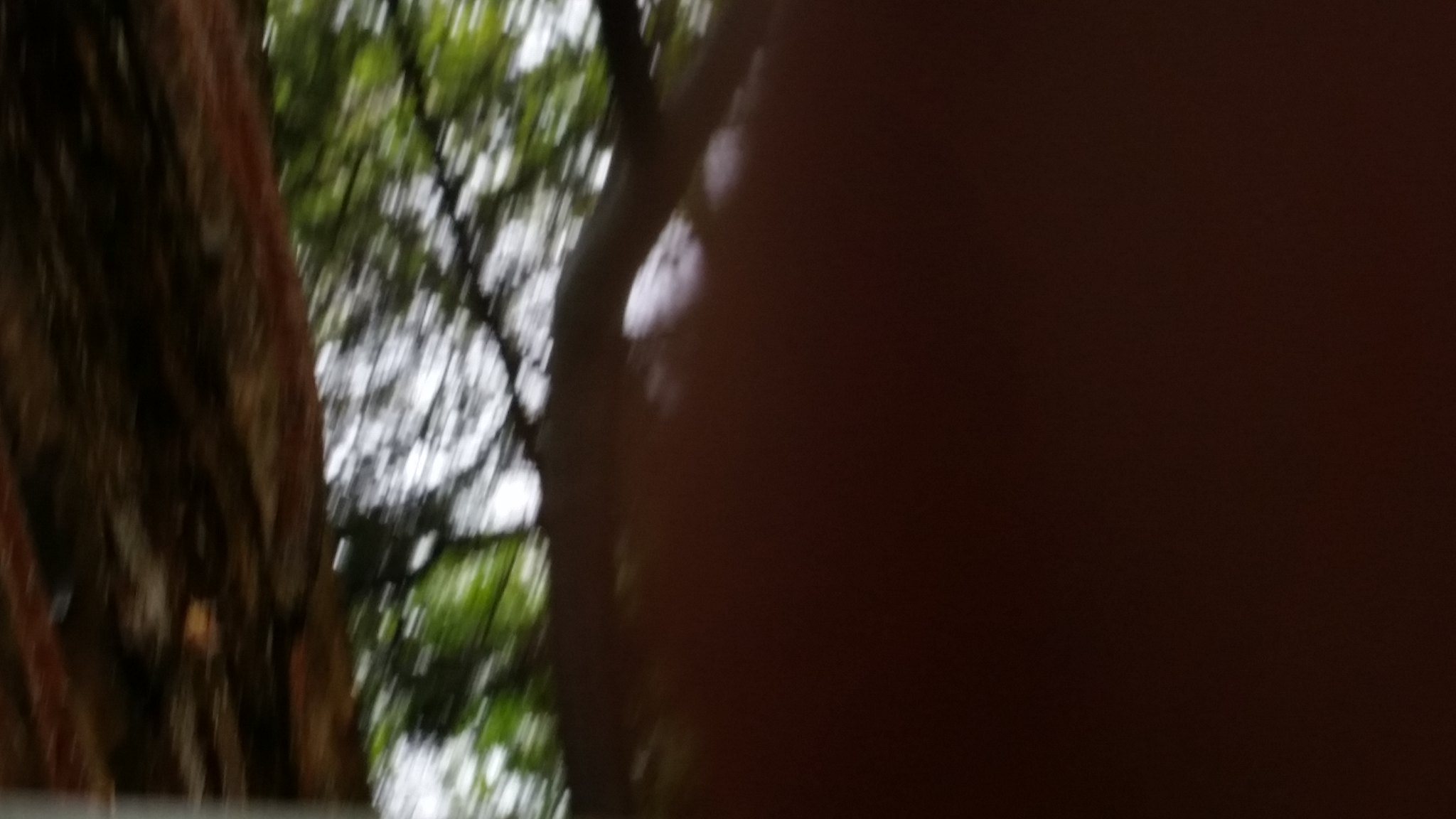This photograph features a dynamic, motion-blurred scene created by moving the camera while the shutter was open. Dominating the right side of the image, a large, dark brown tree trunk takes up nearly two-thirds of the frame. On the left, a slimmer tree trunk occupies about one-fifth of the space. Between these two trunks, a V-shaped gap frames a glimpse of the sky, which appears as a light, vague blur. Surrounding the tree trunks, the blurred lines and patches of green suggest the presence of leaves and branches. The interplay of dark browns from the trunks, greens from the foliage, and the lightness of the sky create an abstract, painterly effect that captures the frenetic energy of the scene.